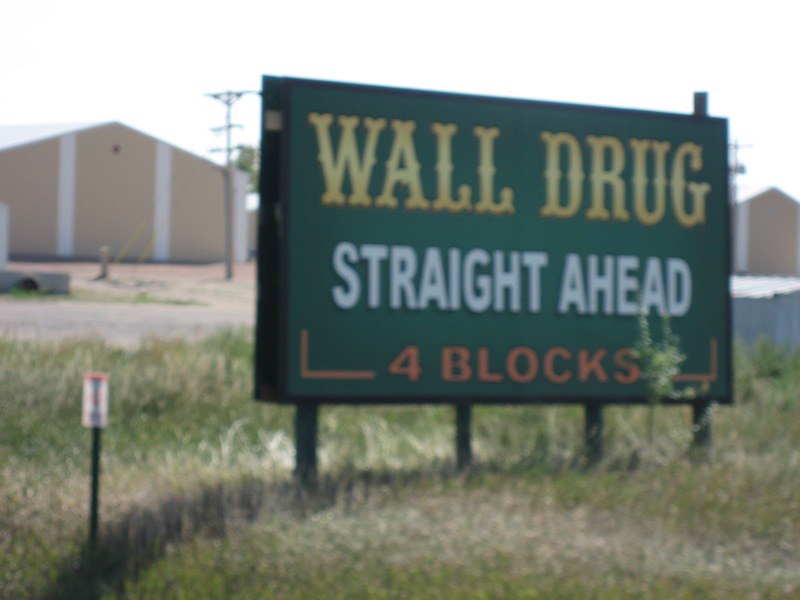The image depicts a large, slightly out-of-focus rectangular sign situated in a rural area, surrounded by wild, overgrown grass, some of which is yellowed and dead. The sign, which is predominantly hunter green, prominently displays the message "Wall Drug Straight Ahead Four Blocks," with "Wall Drug" in yellow letters, "Straight Ahead" in white, and "Four Blocks" in orange. The sign is mounted on four posts and has a noticeable hollow side, consisting of two pieces of wood hanging down. In front of the sign, a big weed is distinctly visible. Nearby, there is a green post with a square white sign at its end, and a pole with a white canister with a red top. The background features beige-colored metal warehouse buildings with white vertical stripes and pointy roofs, along with some electrical poles scattered around.